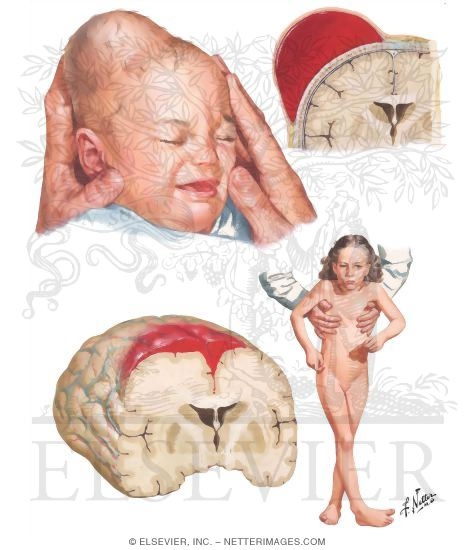Set against a stark white background, the image is divided into four distinct quadrants, each depicting unsettling and bizarre scenes. In the top left, there's an image of a distressed baby with closed eyes and an open mouth, clearly crying. The baby's head appears misshapen with a significant bulge at the back. Two adult hands firmly grasp the baby's head—one touching the right temple, the other supporting the back and under the left ear, emphasizing the abnormality of the skull.

In the top right, a detailed illustration showcases a human brain with an ominous red dome, suggesting a severe medical anomaly like a tumor or hemorrhage positioned atop the brain. The bottom left image mirrors this with a cross-section of a brain, showing a pool of blood seeping into the brain stem, reinforcing the severity of the condition highlighted in the top right quadrant.

In the bottom right, an unsettling depiction features a naked young girl with brown hair, held under her armpits by a man's hands. The girl appears to have an unnatural, almost dazed expression. Her right leg is bent over her left, lending a disquieting and awkward appearance to the scene.

The detailed visuals and repeated emphasis on abnormal growths and distressing figures across the quadrants create a deeply disturbing and eerie overall composition.